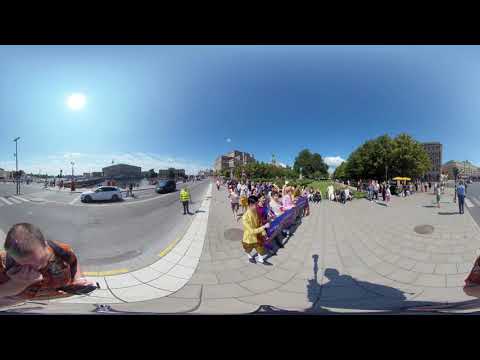This image, taken midday under a clear sky with the sun high overhead, presents the view reminiscent of looking through a peephole, giving it a warped and bent perspective. The photo features a bustling parade scene with numerous people marching down a sidewalk. At the forefront, several women, dressed in a medley of colors including yellow, red, and blue, hold a long, horizontal purple banner. Among them, a notable person at the end of the line wears a yellow long-sleeve jacket. The shadow of an individual centrally located suggests they might be holding a microphone.

The sidewalk on which the parade progresses bends from one street to another, framed by a roadside on the right and a road on the left. To the left, nearer the edge of the image, stands a white car in front of a building, behind a man in the bottom-left corner dressed in an orange shirt. Further into the middle, on the far edge of the road, a man in a yellow vest stands.

In the paraded backdrop, rows of people continue walking, with a park visible behind them featuring grassy areas, trees, and a prominent building in the center. To the right, beyond the parade, another building stands, with more people making their way down the adjacent road. The landscape looks slightly disoriented, as if space itself is contorted and directions are somewhat perplexing due to the warping effect of the image.